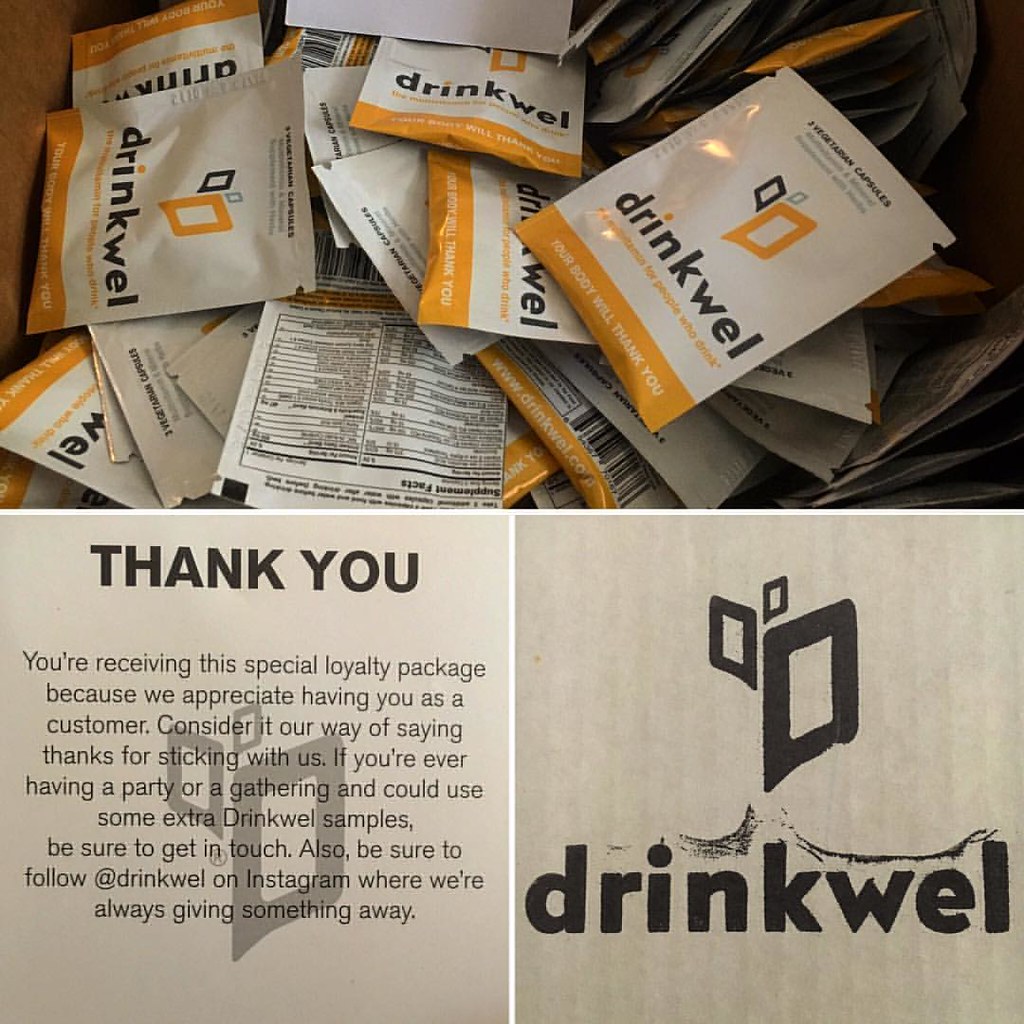The image is a promotional advertisement featuring a product called "Drinkwel," which appears to be health or wellness supplements designed to be added to beverages. The top half of the image prominently displays several individual packets labeled "Drinkwel," each package white at the top with a centered logo consisting of three semi-diamond shapes—orange, black, and gray—in decreasing sizes. The packets also bear the name "Drinkwel" in brown font and some text suggesting it says "Body Well Thank You," alongside visible but unreadable nutritional information due to small print on one flipped packet. The bottom half of the image is divided into two sections: the right side shows the Drinkwel logo against a gray background with the text "Drinkwel" in dark gray font, and the left side features a bold "Thank You" note in uppercase with additional text explaining that the recipient is part of a special loyalty program. This note extends gratitude for their loyalty, encourages them to follow @drinkwel on Instagram for giveaways, and hints at potential additional perks for parties or gatherings.